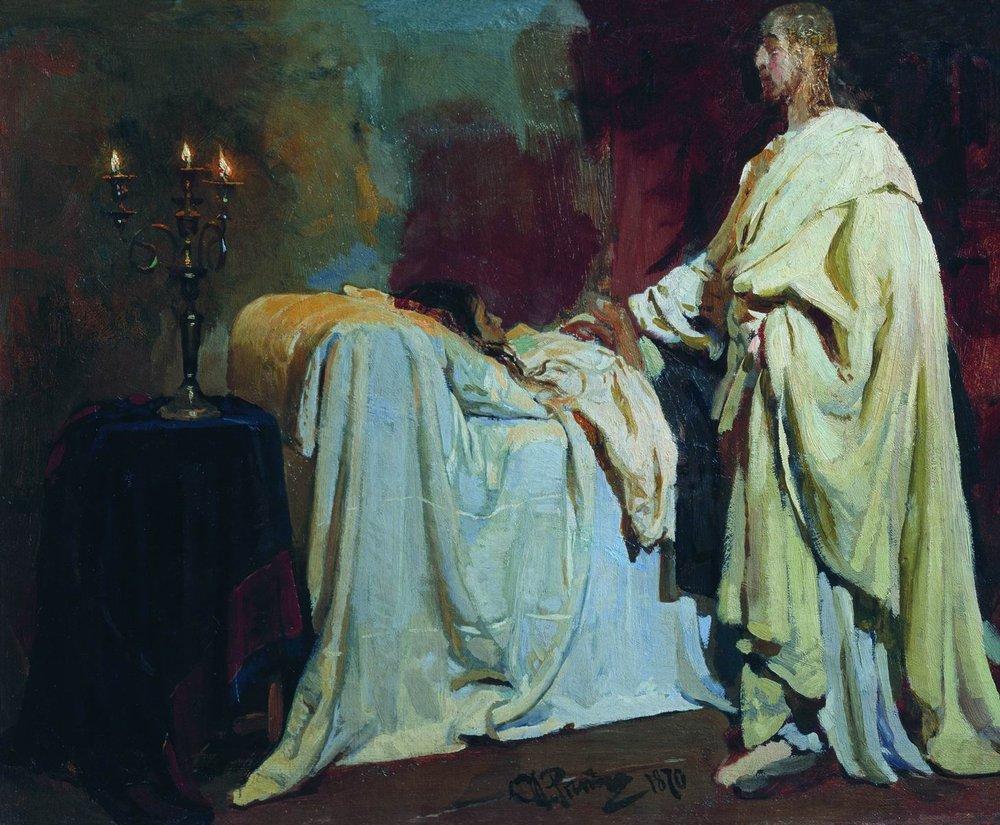The realistic painting depicts a biblical scene, likely the healing of Jairus' daughter by Jesus. Dominating the right side of the image is a figure of Jesus, robed in layers of primarily green, light yellow, and blue garments, his brown hair cascading to his shoulders, framing a brown beard. His left shoulder and right arm are draped in white, with his right hand stretched out over a sick girl lying in an elevated bed covered with white sheets and blankets. The girl, with her black hair and faint profile visible, has her hands placed on her stomach. To the left of the bed stands a wooden table draped in a deep blue, velvety tablecloth with purple edging, upon which a black metal candelabra with three lit flames is situated. The setting appears to be a dimly lit bedroom, characterized by an intricate blend of dark hues including blues, oranges, reds, yellows, and blacks that create a dramatic and somber atmosphere. The floor seems wooden, adding a rustic feel to the scene.